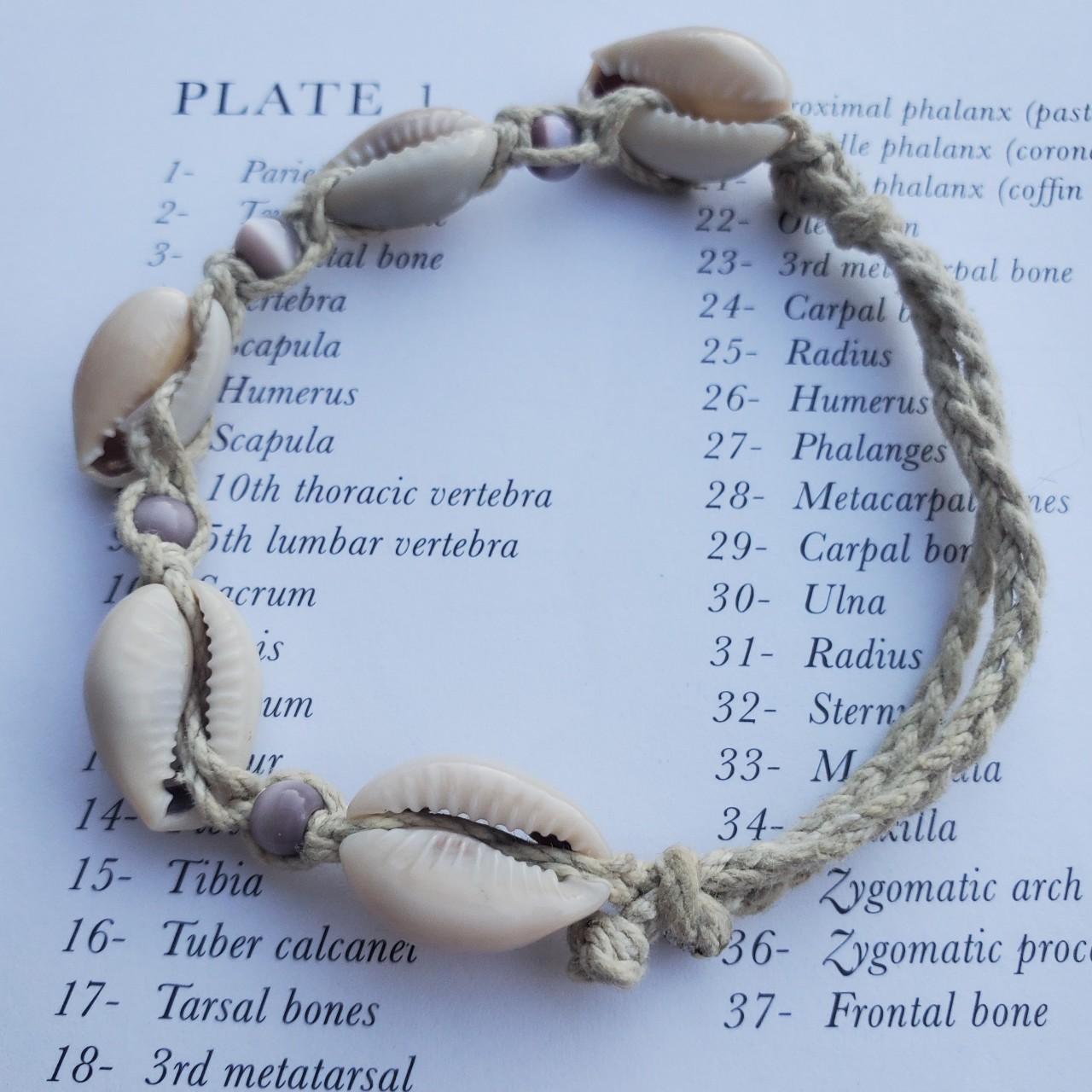This image features a detailed close-up of a braided natural-toned bracelet that looks like a henna rope bracelet. The bracelet is adorned with five seashells in varying shades of white, cream, and gray, and four round magenta beads are interspersed among the shells. The background consists of a light blue piece of paper that displays text in black. The heading on the top left reads "Plate 1." The text includes names of various body parts such as humerus, phalanges, metacarpals, carpal, ulna, scapula, 10th thoracic vertebra, vertebrae, tibia, tarsal bones, and the 3rd metatarsal, with numbers running sequentially down the side from 1 to 37, some of which are partially obscured by the bracelet.